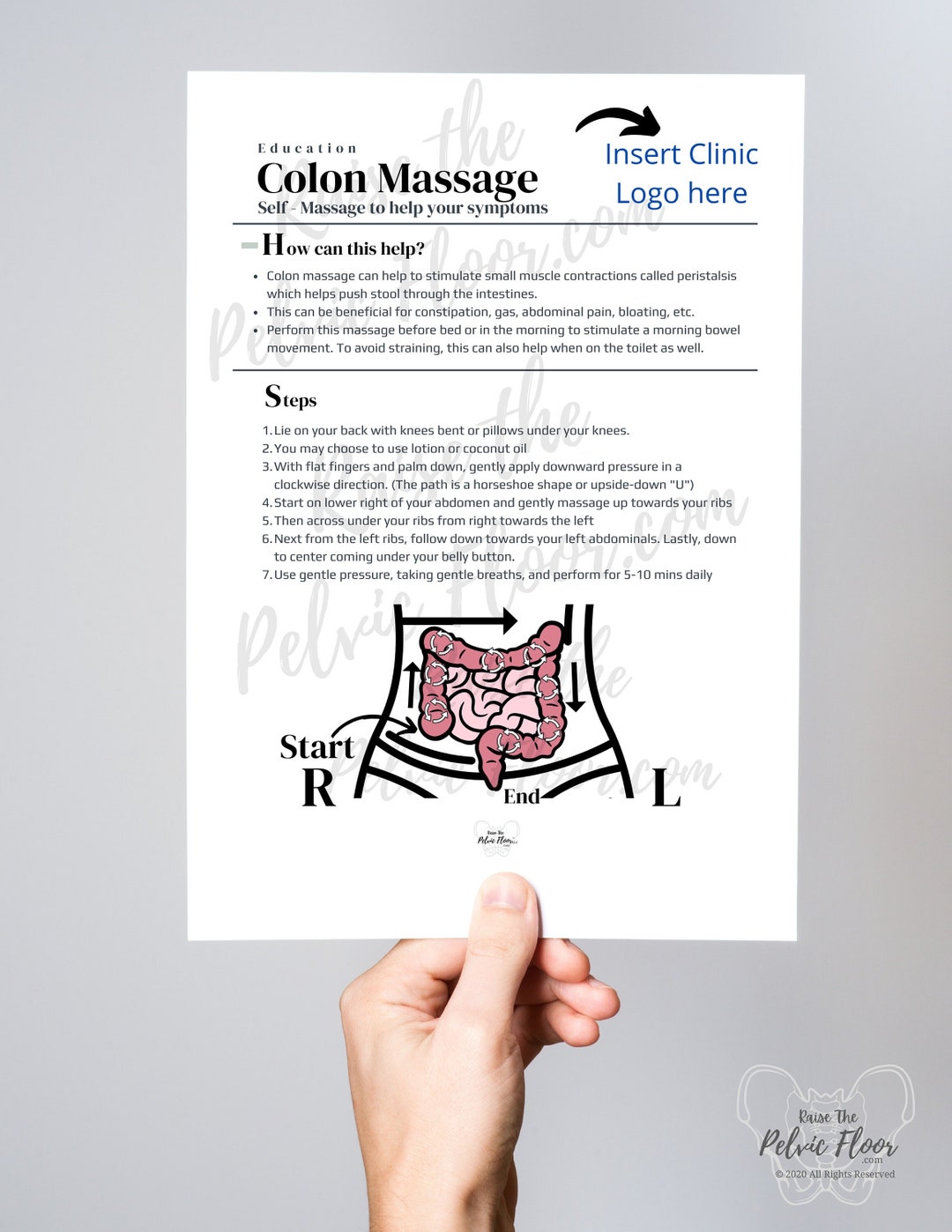The image features a white person’s hand holding a white sheet of paper designed as an infographic for various clinics, primarily for medical purposes. At the top left of the sheet, it reads "Education: Massage" in bold black letters, followed by "Self-massage to help your symptoms" in smaller black letters underneath. To the upper right, there is a black arrow pointing to blue text that says "Insert Clinic Logo Here." The infographic includes detailed instructions on how to perform a colon massage, explaining its benefits and the steps involved. The lower section of the sheet prominently features a colored illustration of the human intestines, depicted in a pinkish hue, contrasting with the predominantly black text on the white background. Additionally, the lower right part of the infographic is watermarked with "pelvichome.com." The overall design is both informative and visually accessible, making it an effective educational tool for patients.